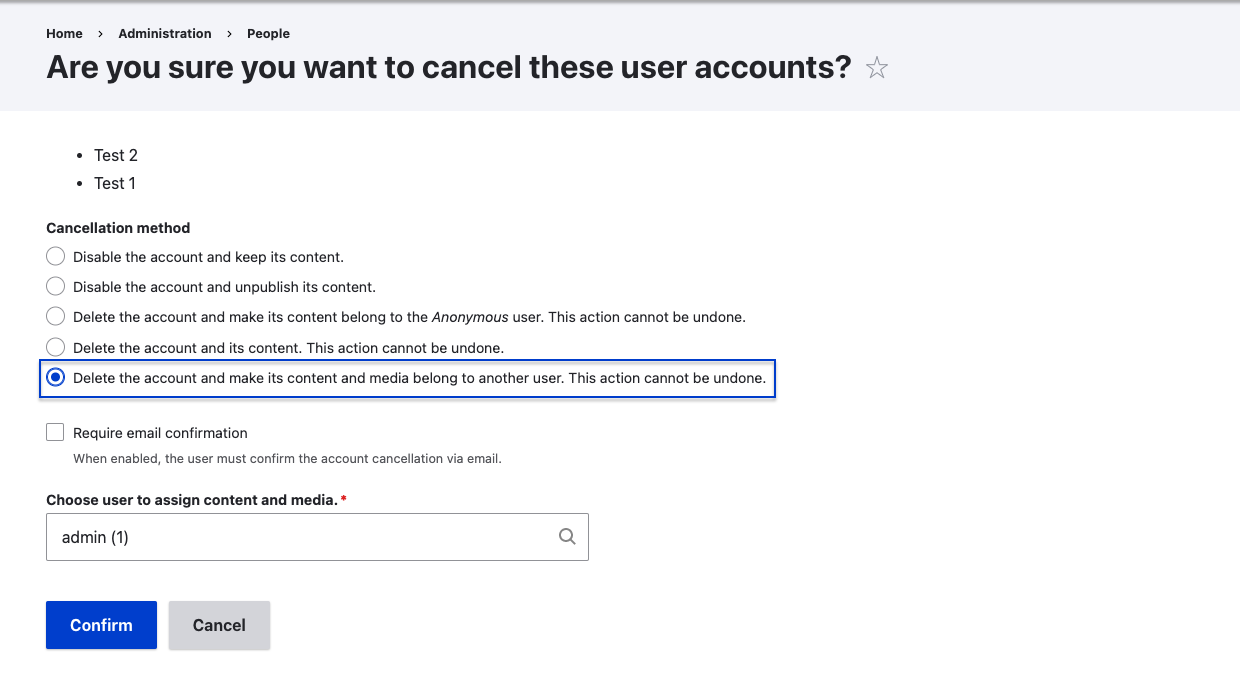Screenshot from a website interface:

At the top of the screenshot, there is a light gray background with black text, indicating the current section of the website as "Home > Administration > People." The headline reads, "Are you sure you want to cancel these user accounts?"

Below the headline, there are two bullet points listing the user accounts to be canceled: "test2" and "test1."

Following the list of users, there is a bolded title that says "Cancellation method." Under this title, a variety of account cancellation options are provided:

- Disable the account and keep its content.
- Disable the account and unpublish its content.
- Delete the account and make its content belong to the anonymous user. This action cannot be undone.
- Delete the account and its content. This action cannot be undone.
- Delete the account and make its content and media belong to another user. This action cannot be undone. 
The last option is currently selected.

Additionally, beneath these options, there is a checkbox labeled "Require email confirmation." This option specifies that the user must confirm the account cancellation via email if enabled.

Finally, there is a section titled "Choose user to assign content and media," which appears because the selected option is to delete the account and reassign its content and media to another user.